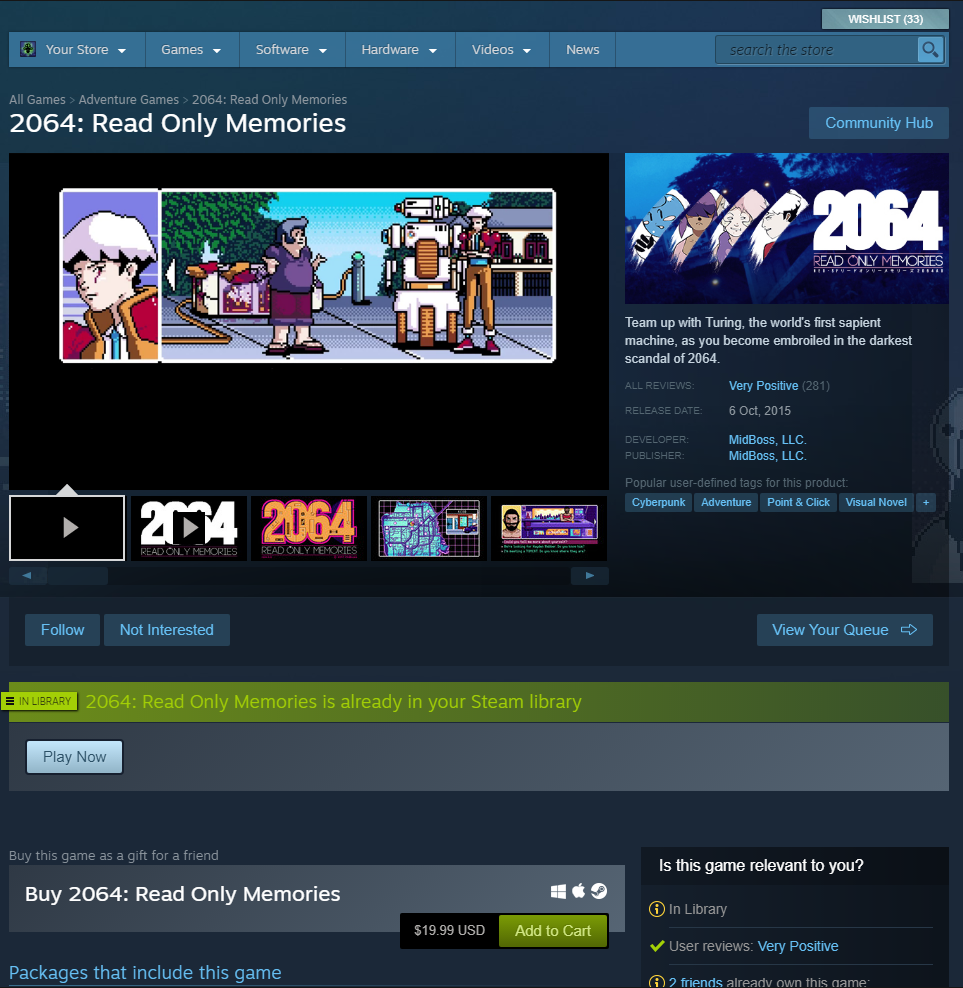The image portrays a website interface, potentially a platform focused on gaming. The top section features several navigation tabs labeled as "Store," "Games," "Software," "Hardware," "Videos," and "News," each accompanied by a dropdown arrow. Above these tabs, there is a "Wish List" option, and below, a prominently placed search bar with the placeholder text "Search the store."

Centered on the page is a colorful, pixelated graphic depicting two men standing beside what appears to be a robot. This image is headlined with the title "2064: Read-Only Memories," which is repeated in an adjacent box. Below the main image, there are additional thumbnail images suggesting other selections or related content. 

To the side, there are interactive buttons labeled "Follow" and "Not Interested," and towards the bottom of the interface, a "Play Now" button is visible, accompanied by an "Add to Cart" option for seamless purchasing.